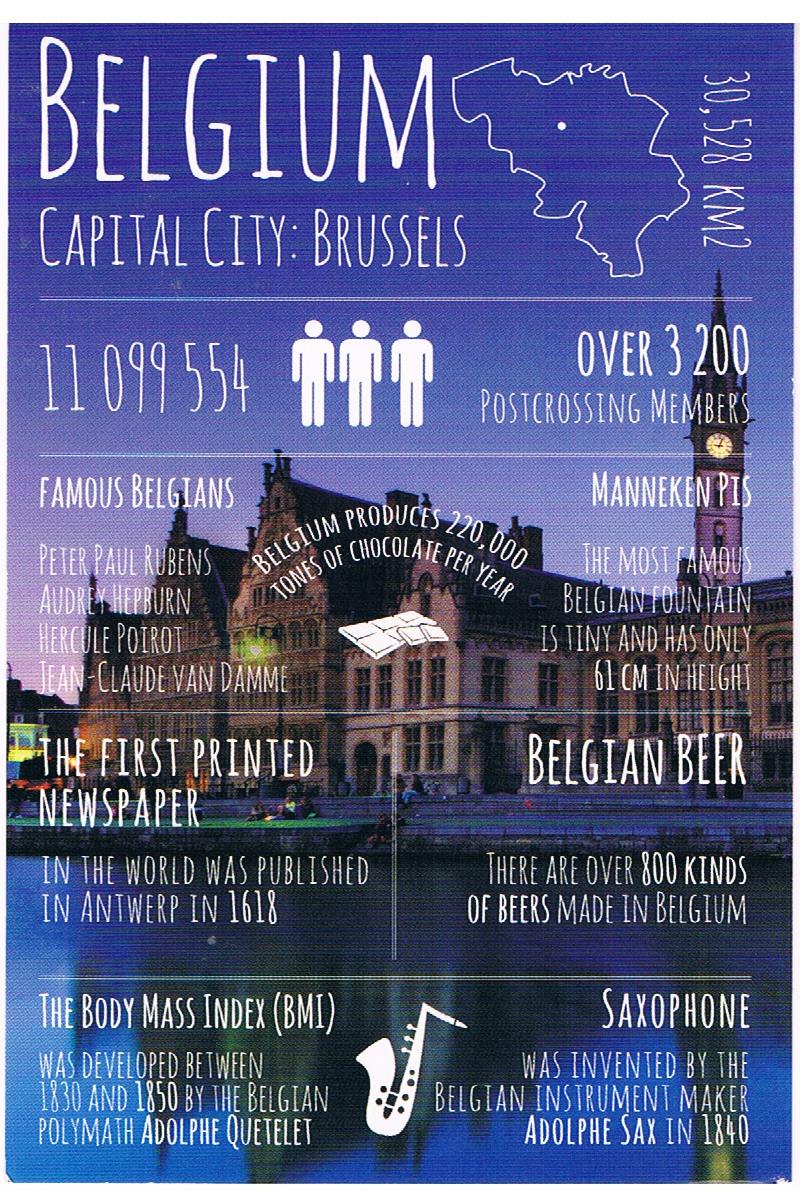This image features a detailed poster promoting Belgium. The centerpiece is a tall brick building, possibly a church with a clock tower, set against a purple-hued sky, reflected in a tranquil body of water in the foreground. People are sitting on the steps near the water, and a boat is visible to the left. At the top of the poster, "Belgium Capital City Brussels" is prominently displayed, accompanied by a map showing Belgium's outline with Brussels marked by a dot. To the right, the country's area of 30,528 km² and population of 11,099,554 are noted alongside three iconographic stick figures. Below, the poster highlights Belgium's cultural and historical significance, mentioning that the BMI (Body Mass Index) was developed there, the saxophone was invented in 1840, Belgium produces 220,000 tons of chocolate per year, and it is well-known for its beer. Other facts include the printing of the first newspaper in Belgium and a roster of famous Belgians like Peter Paul Rubens. The poster also states there are over 3,200 post-crossing members in the country.